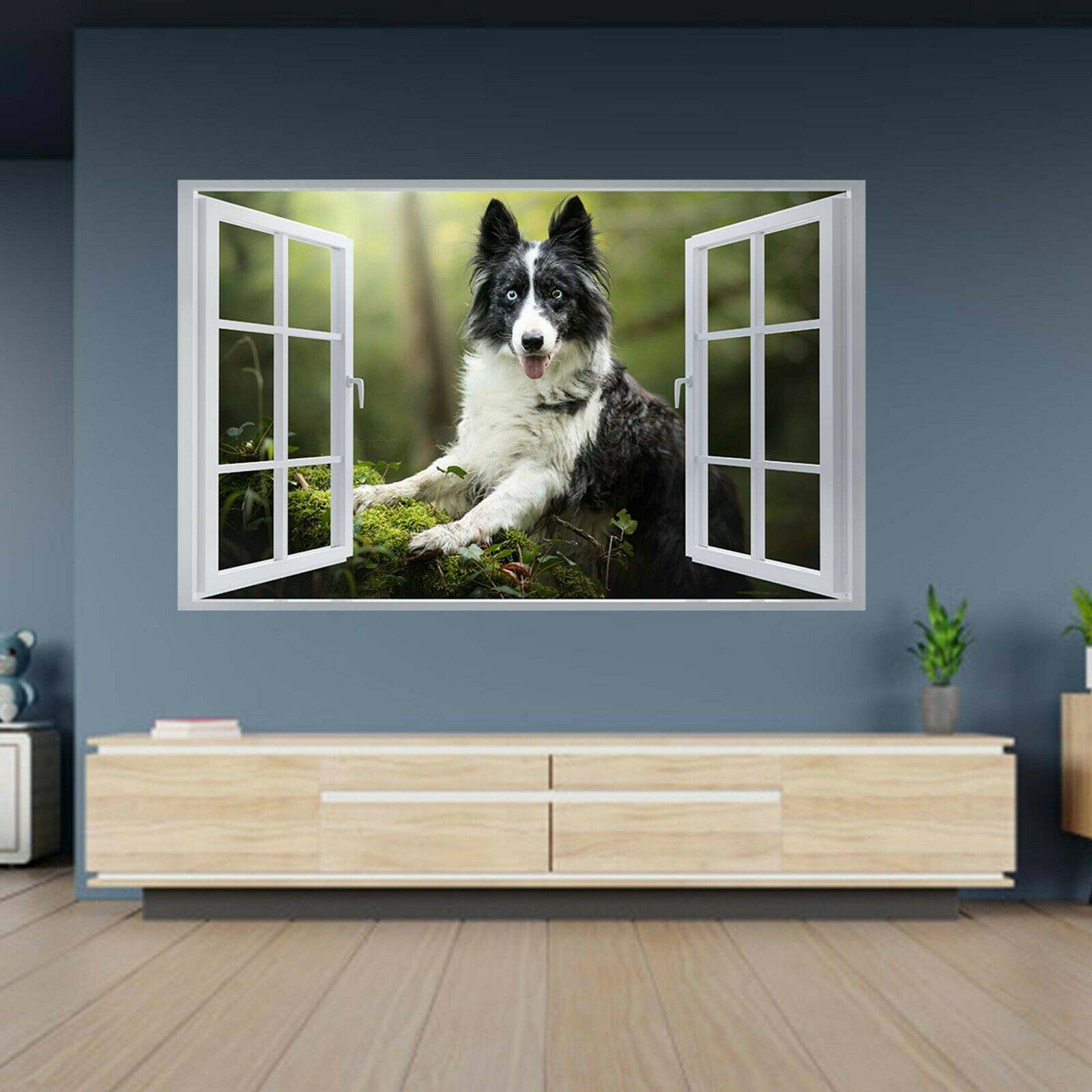The photograph captures a detailed image of a black and white dog standing on its hind legs. The dog, which appears to be a smaller breed with a fluffy tail, showcases mostly black fur on its face and back, while the front part is predominantly white. The distinct markings include a white stripe from the top of its nose to the back of its head, and its bright blue eyes add a striking contrast. The dog stands in front of a large, dark-framed, multi-pane window that seems to open onto a green solarium area.

The setting of the photograph appears to be an indoor space, possibly an office, living room, or lobby with navy blue or white-blue walls. Below the window, there is a wooden entertainment center or table stained a light brown, with a couple of books on the left side and a green, succulent-like plant in a gold vase on the right. The floors are made of long vertical wooden slats, stained a light brown. There is a small table to the left with a ceramic bear and, in the background, a white surface with a blue teddy bear on it is visible. The overall composition gives a cozy and inviting feel to the space.